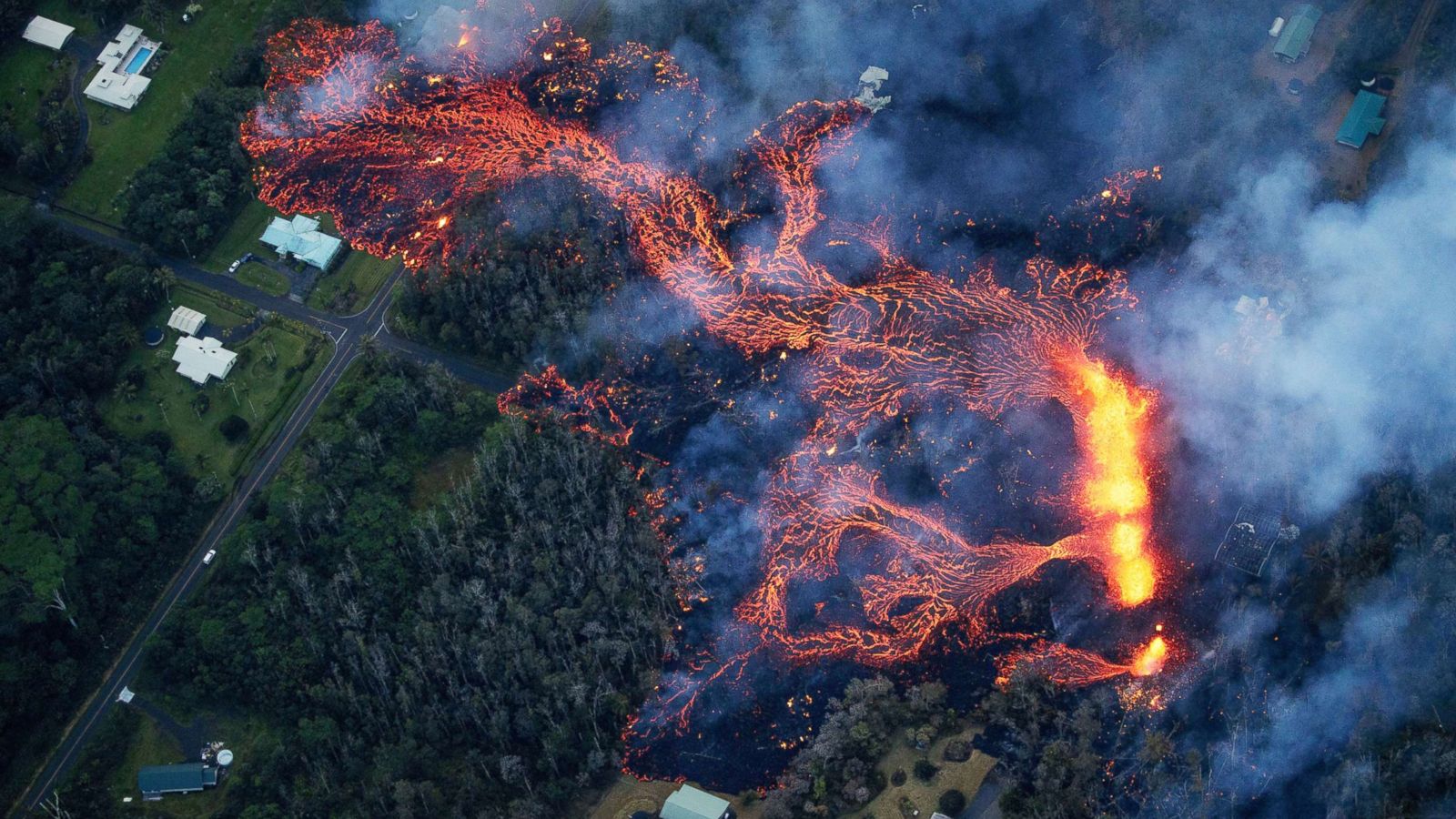This aerial view captures a dramatic and devastating forest fire unfolding over a landscape divided into distinct sections. On the left side, dense greenery with tall trees interspersed with buildings and a small house dominate the scene. A road with a few cars cuts through this lush before opening up into more grassy areas and a cluster of three white houses. The afternoon light casts a somber tone over the area.

On the right side, the picture reveals a stark contrast as thick black and gray smoke billows up, with trails of both white and ash-colored smoke swirling around. The inferno's molten, lava-like fire spreads methodically across the middle and right side of the image, seeping ominously into the untouched green areas. The relentless flow of lava and towering flames are depicted pouring from an orange glow, spelling imminent destruction for the lush forest below. Trees are clearly succumbing to the heat, burning and disintegrating as the fire stretches across multiple blocks. The scene, captured from a high angle, underscores the breadth and intensity of the calamity, illuminating the full scale of its devastating impact.